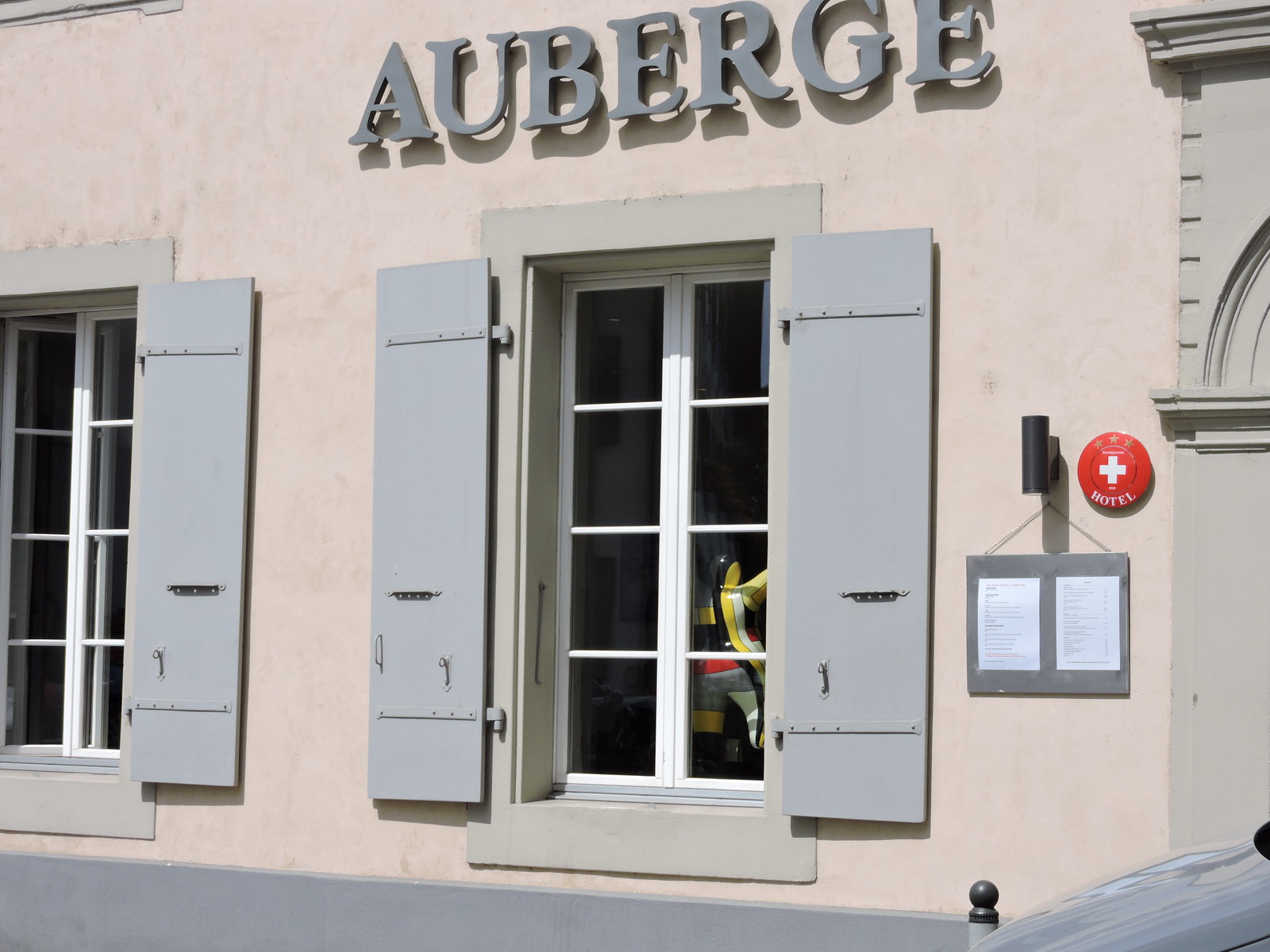The image captures the front view of a light cream-colored building. Prominently displayed at the top center is the word "AUBERGE" in gray letters, which slightly protrude from the wall, creating a reflective shadow. Beneath the text is a window featuring an eight-pane white frame, encased in a light gray square. This window is flanked by open gray shutters. Visible through the window is a stylized statue of a man, crafted from yellow, black, white, and gray clay. To the immediate right of the window, a black sconce lamp extends from the wall with a wire connecting to a gray square, bookended by two white pieces of paper. Just above and adjacent to this is a red circular sign with a white cross, labeled "Hotel" in white text, topped by three gold stars. A gray horizontal line runs along the bottom of the building, and in the bottom right corner, the shiny hood of a gray car with a rusty-colored hitch is partly visible.